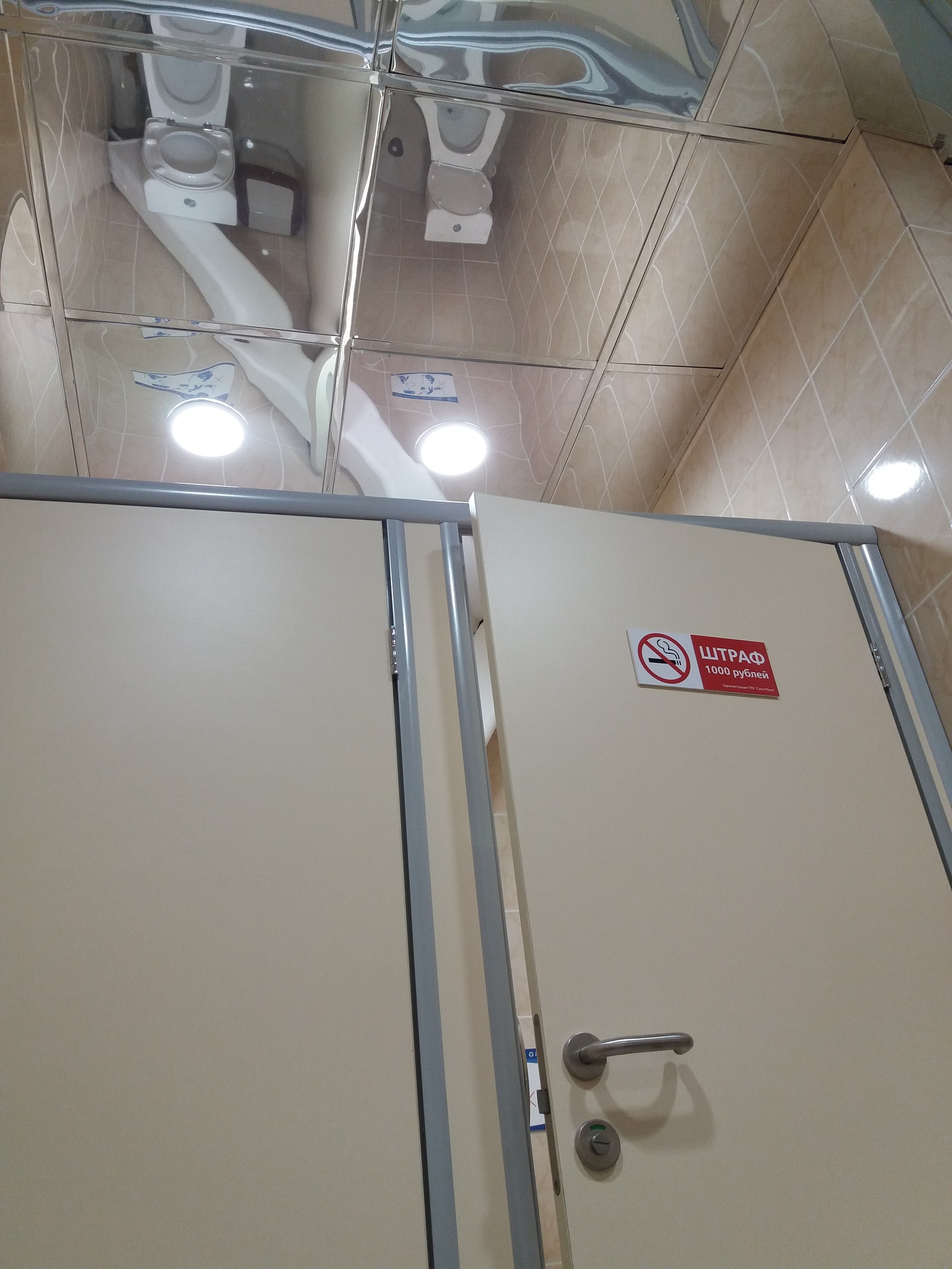This photograph captures an unusual bathroom scenario, likely taken in a foreign country given the non-English logos on signs. The image is in portrait orientation, showcasing a low, upward angle, perhaps taken from the floor or by a very short individual. This perspective places the viewer close to door-handle level. The focal point includes two adjacent, bright yellow bathroom doors, framed by a yellow border and set within a sleek gray frame. These doors are mounted against a modern, beige tile wall.

A perplexing feature of this bathroom is the ceiling, which is fully mirrored, an unconventional choice for any setting, let alone a restroom. This unusual addition allows a clear overhead view into the stalls, infringing on the privacy typically afforded by bathroom doors. This design choice is both intrusive and inefficient, as it compromises the discretion that individuals expect and deserve while using such facilities.